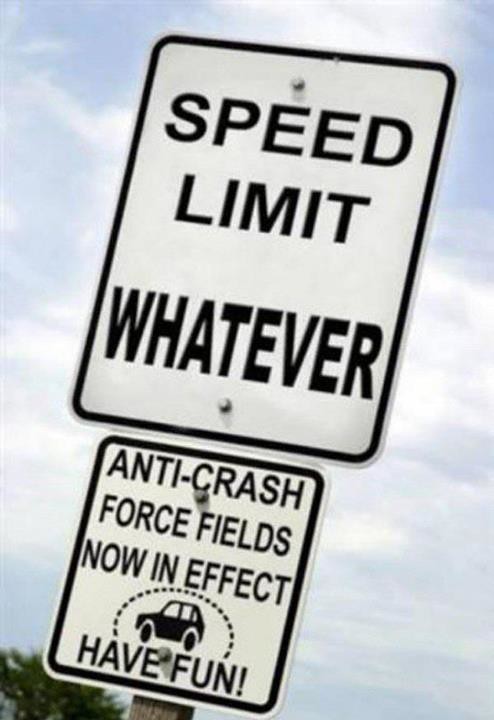This is a photograph of two humorous road signs stacked on a wooden pole, photographed against a hazy, lightly cloudy blue sky during daytime. The image is slightly blurry and taken from a slanted, lower angle, giving a view of the signs from below. The top sign mimics a typical American speed limit sign but humorously reads "Speed Limit Whatever" instead of displaying a number. Below it, a smaller sign states, "Anti-Crash Forcefields Now in Effect, Have Fun," accompanied by a whimsical illustration of a car encircled by a dotted line, suggesting a protective force field. A bit of foliage from a treetop is visible in the bottom left corner, hinting that the photograph is likely edited as part of a satirical meme. The signs stand out with their white backgrounds, black borders, and black text, creating a stark contrast against the sky. The photograph itself is medium in quality, measuring approximately five inches wide by eight inches tall, and lacks any borders.